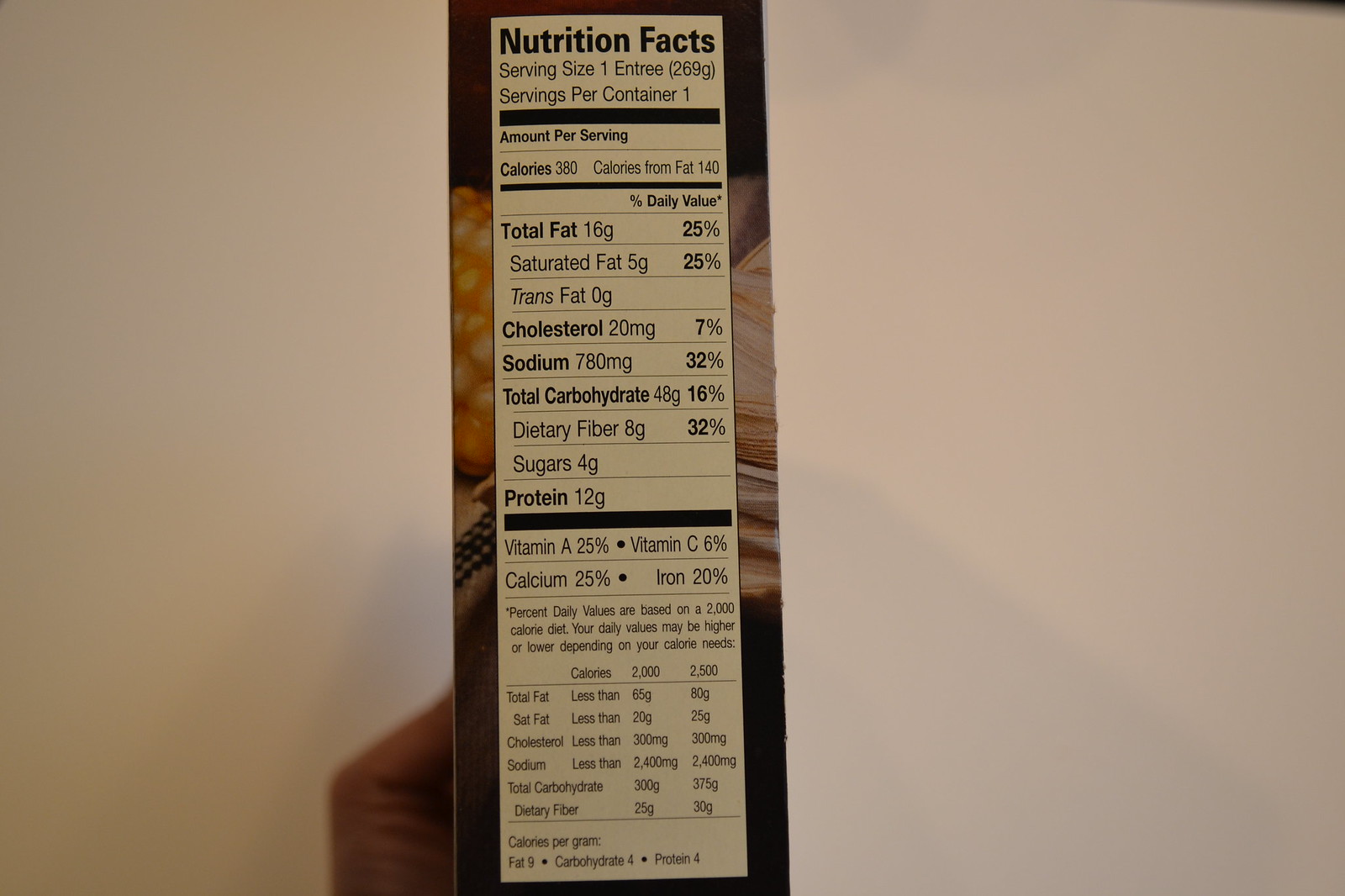The image is a color photograph of a nutrition label on a food container, which is being held up by someone’s hand. The photograph centers on the nutrition label, which is a long, thin, off-white rectangle with black lettering. The background is a beige-peach color, possibly under indoor lighting or dim sunlight. The person's hand is visible at the bottom left, and a faint shadow is cast behind the hand. There's a black border at the top and bottom of the label, framing it within the container. To the sides of the label, there are indistinct pictures of food in brown, cream, and orange hues, with possibly corn visible on the left.

The nutrition label lists detailed dietary information including a serving size of one entree (269 grams), with one serving per container. It specifies the calories as 380, with 140 calories from fat. The total fat content is 16 grams, saturated fat is 5 grams, and trans fat is 0 grams. The label also mentions 20 milligrams of cholesterol, 780 milligrams of sodium, 48 grams of total carbohydrates, 8 grams of dietary fiber, 4 grams of sugars, and 12 grams of protein. Additionally, it includes percentages for vitamin A, vitamin C, calcium, and iron based on daily recommended values.

Below the main nutritional information are further details that include black horizontal bars separating sections. These sections cover various nutritional contents and also provide a table with daily values for total fat, cholesterol, sodium, and total carbohydrates based on a 2,000 and 2,500 calorie diet. The fine print at the bottom contains additional information that is too small to read clearly. Overall, this detailed descriptor conveys thorough nutritional information and suggests the food product might not be particularly healthy due to its fat, cholesterol, and sodium content.